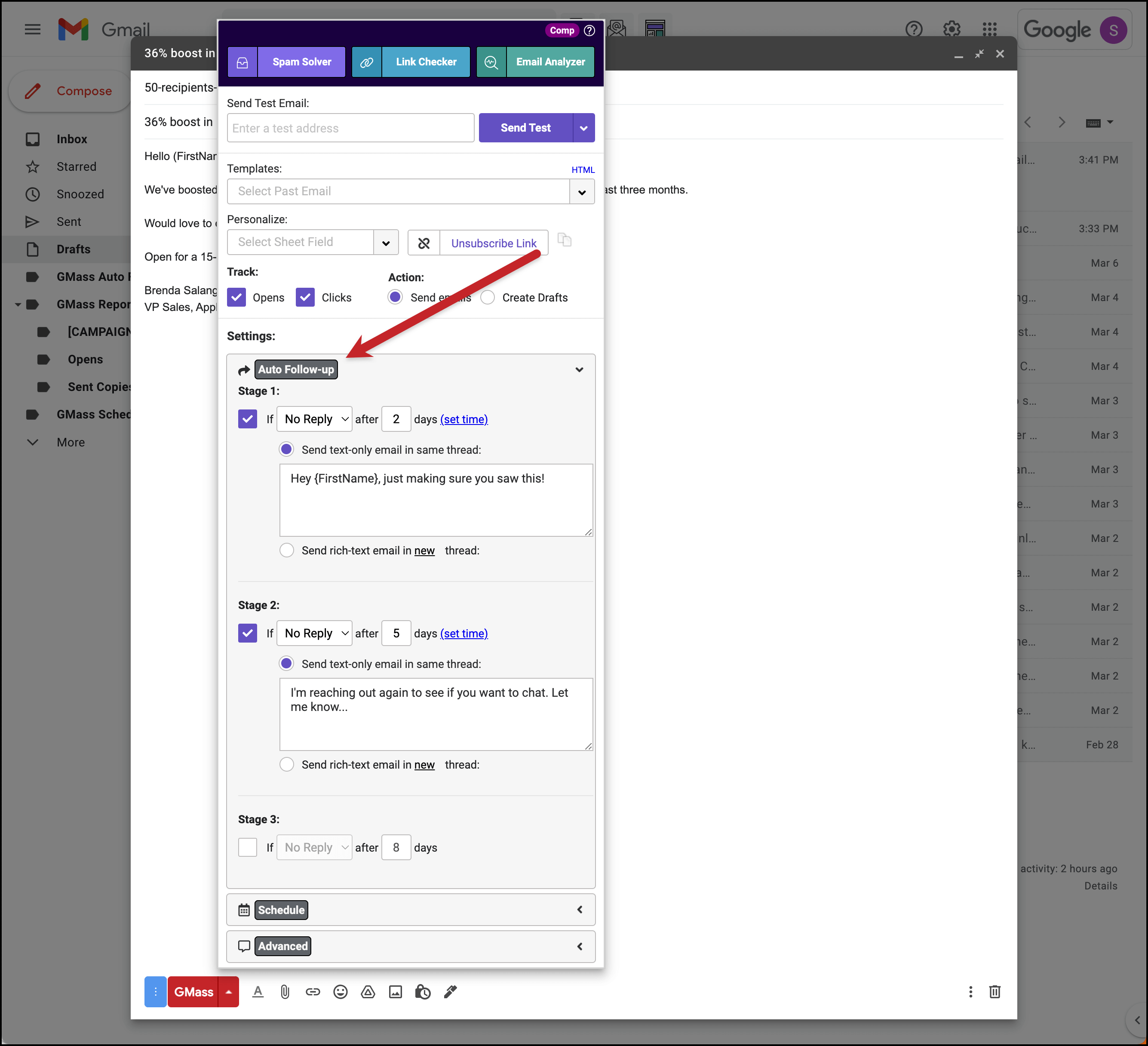The image depicts a Gmail interface on a gray background, divided into two sections. The left side houses a menu, while the right side contains a list that is grayed out, making it unreadable. Two pop-up windows obscure the central content. 

The larger pop-up window contains text that is too small to decipher and remains unreadable even after attempts to zoom in and out. Overlapping this window is a smaller one, which prominently features three colored boxes at the top: a purple box on the left, a blue box in the middle, and a dark green box on the right. Below these boxes is a text box. To the right of this text box is a purple button with a drop-down menu. Directly beneath it is another text box, followed by a smaller text box. Underneath these are several lines of text accompanied by checked checkboxes. 

A black rectangular shape with some text inside it appears at the bottom of this smaller window. A red arrow pointing downwards directs attention to this black rectangle.